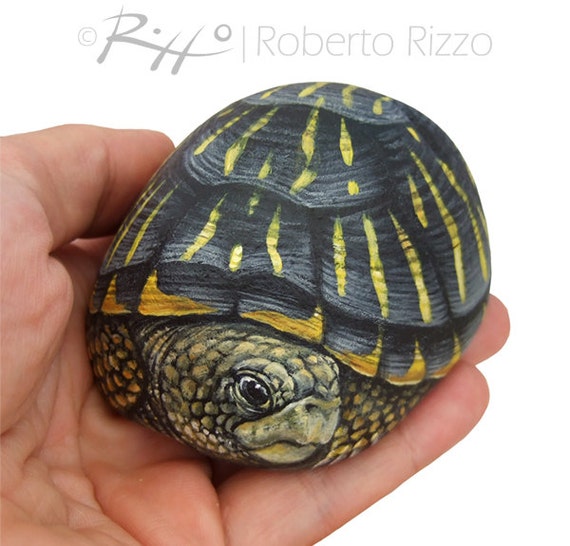In this image, a painted rock is being held in the left hand of an individual, with the hand positioned palm-upcoming from the top left of the frame. The rock has been intricately painted to resemble a detailed turtle. The turtle's shell is predominantly gray with streaks of yellow running across it, giving it a dynamic, textured appearance. The turtle’s body, also in shades of gray, features yellow blotches and an intricate scaly texture, particularly around the arms which are tucked in by its sides, creating a lifelike effect.

The turtle's head, characterized by its beak-like shape, light grayish-green tone, and delicate features such as oval eyes with prominent black pupils and small nostrils, is poking out and looking towards the bottom right of the image. The shell extends towards the top right, contrasting with the head's direction. Above the image, there is a logo in gray lettering that reads "© RH | Roberto Rizzo," with "RH" stylized in a calligraphic script and "Roberto Rizzo" presented in a thin font.

The image captures a moment of curiosity and craftsmanship, emphasizing the highly detailed and realistic portrayal of the turtle on the rock, attributed to the artist, Roberto Rizzo.